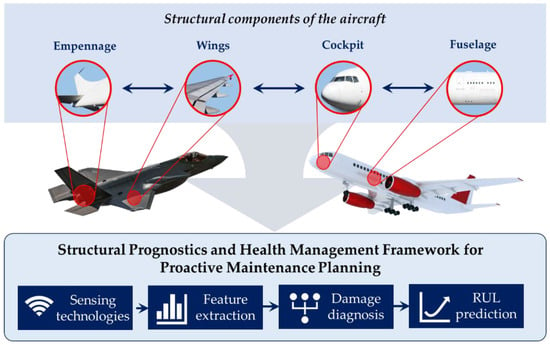This diagram is an illustrative infographic about aircraft components and a structural health management framework. The top section features a light blue banner labeled "Structural Components of the Aircraft." It includes four red-bordered circles that illustrate and label the empennage, wings, cockpit, and fuselage, each with red arrows pointing to corresponding sections on two depicted airplanes. One airplane is a military-style dark gray jet on the left, while the other is a commercial passenger-style white jet on the right. Both airplanes are oriented towards each other and slightly upwards. The central portion of the diagram has a light gray arrow on a white background, pointing down towards the bottom section. Here, a light blue banner reads, "Structural Prognostics and Health Management Framework for Proactive Maintenance Planning," followed by four navy blue boxes labeled sensing technologies, feature extraction, damage diagnosis, and RUL prediction, each box decorated with representative icons.